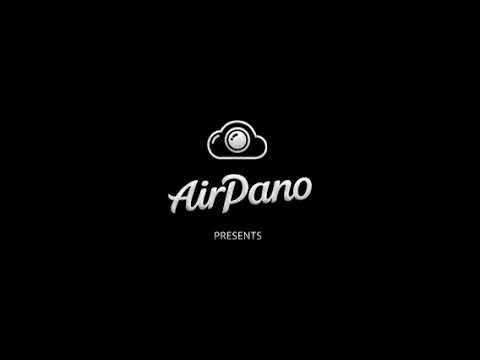The image is a stark, minimalistic design featuring a solid black background with a central white icon. The icon, cartoonish in nature, resembles a cloud with a camera lens embedded in it. This cloud has three humps, creating a somewhat lumpy appearance. Positioned below the icon in a cursive-like font is the word "AIRPANO," written in capital letters as A-I-R-P-A-N-O and appearing as one word. Beneath "AIRPANO," in smaller, thinner all-caps letters, is the word "PRESENTS." All text and graphics maintain a consistent white color. The overall effect suggests that this is a title screen or introductory frame likely for a digital video or production from AIRPANO, potentially indicating the company's involvement in the creation of digital content, such as movies or commercial clips.